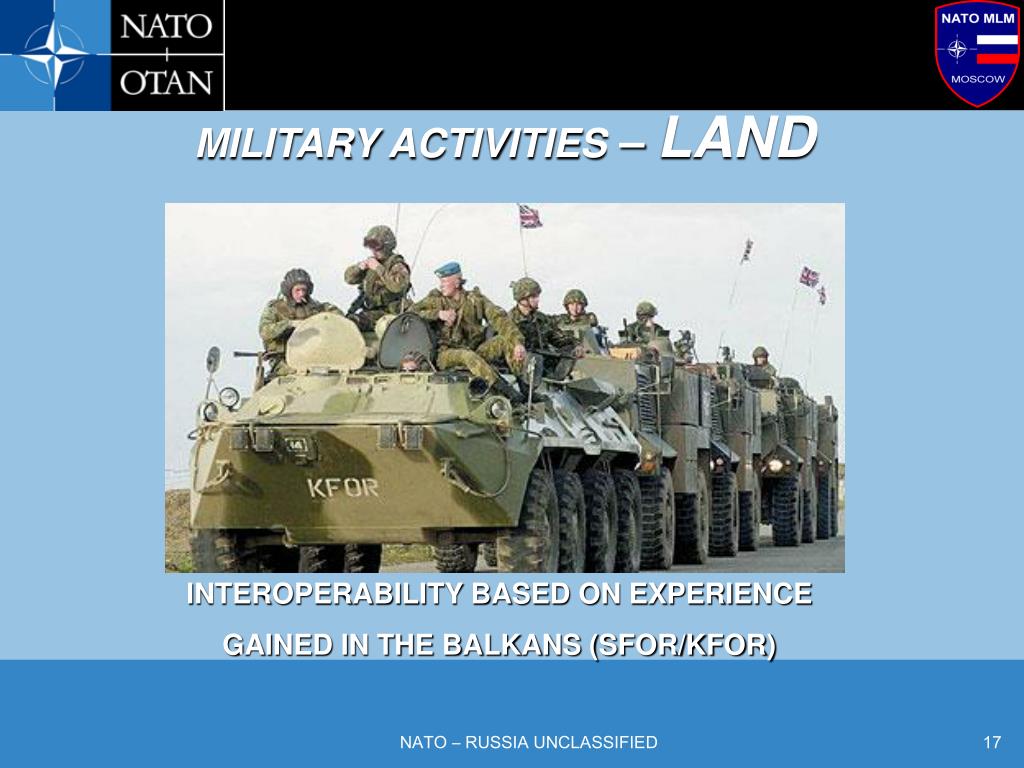The image appears to be a slide from a PowerPoint presentation about NATO military activities. In the upper left corner, there is a logo featuring a pointed star in two shades of blue: navy and sky blue, with the text "NATO" and "OTAN" below it in white lettering on a black background. The upper right corner contains another logo reading "NATO MLM" encased in a shield, with a flag on the right side. The background of the slide is primarily sky blue with a medium blue bar at the very bottom. At the top of the sky blue section, "Military Activities-Land" is written in white, uppercase letters, with the word "Land" in a larger font. In the center, there is an image of military soldiers clad in camouflage uniforms and helmets, riding in a convoy of open-top camouflage vehicles. Below this image, white text reads, "Interoperability based on experience gained in the Balkans (SFOR/KFOR)." At the bottom, additional text says, "NATO-Russian Unclassified," with the number "17" in the bottom right corner. The entire center image is bordered in blue, and the overall presentation emphasizes NATO's military experiences and cooperative endeavors in the Balkans.